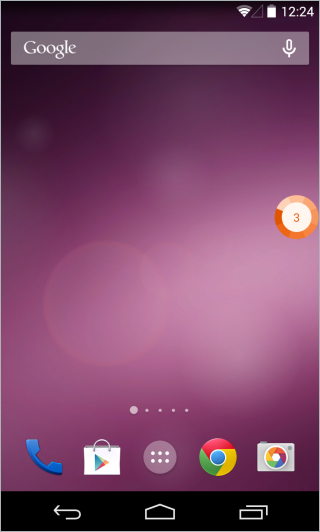A detailed screenshot of an Android smartphone interface, highlighting various elements on the home screen. The background features a gradient of dark purple to black, with lighter purple bubbles scattered throughout, creating a whimsical atmosphere. 

At the top of the screen, there is an almost opaque, white floating rectangle with "Google" boldly written in white on the left side and a white microphone icon on the right, indicating a search bar. Adjacent to this bar, the top-right corner displays a WiFi symbol with three of its four bands lit up, a fully charged battery icon, and a time display reading 12:24 in military time format.

Central to the image is an orange circular widget with a gradient that transitions from dark to light orange, housing a smaller white circle with an orange number "3" inside. 

Near the bottom of the screen, several app icons are arranged. On the far left is the blue and dark blue icon for the calling app. Next, a Google Play Store icon depicted as a multicolored triangle within a white shopping bag. Following this is a circle with six dots (three on the top row, three on the bottom), designated for navigating the app drawer. Above this, five ellipses indicate multiple home screen pages, with one ellipse highlighted by a white circle denoting the current page.

Among the apps, there's also the Google Chrome icon, characterized by thirds of green, red, and yellow forming a circle with a white and blue center. Additionally, a dark grey folder icon containing a multicolored circle reminiscent of a color wheel sits nearby. The circle transitions through colors starting with yellow, orange, burnt orange, red, dark blue, and green, centered by white.

The bottom bezel of the phone shows a navigation bar with a white arrow pointing left for back, a home symbol, and two rectangles for overview of open windows or recent apps.